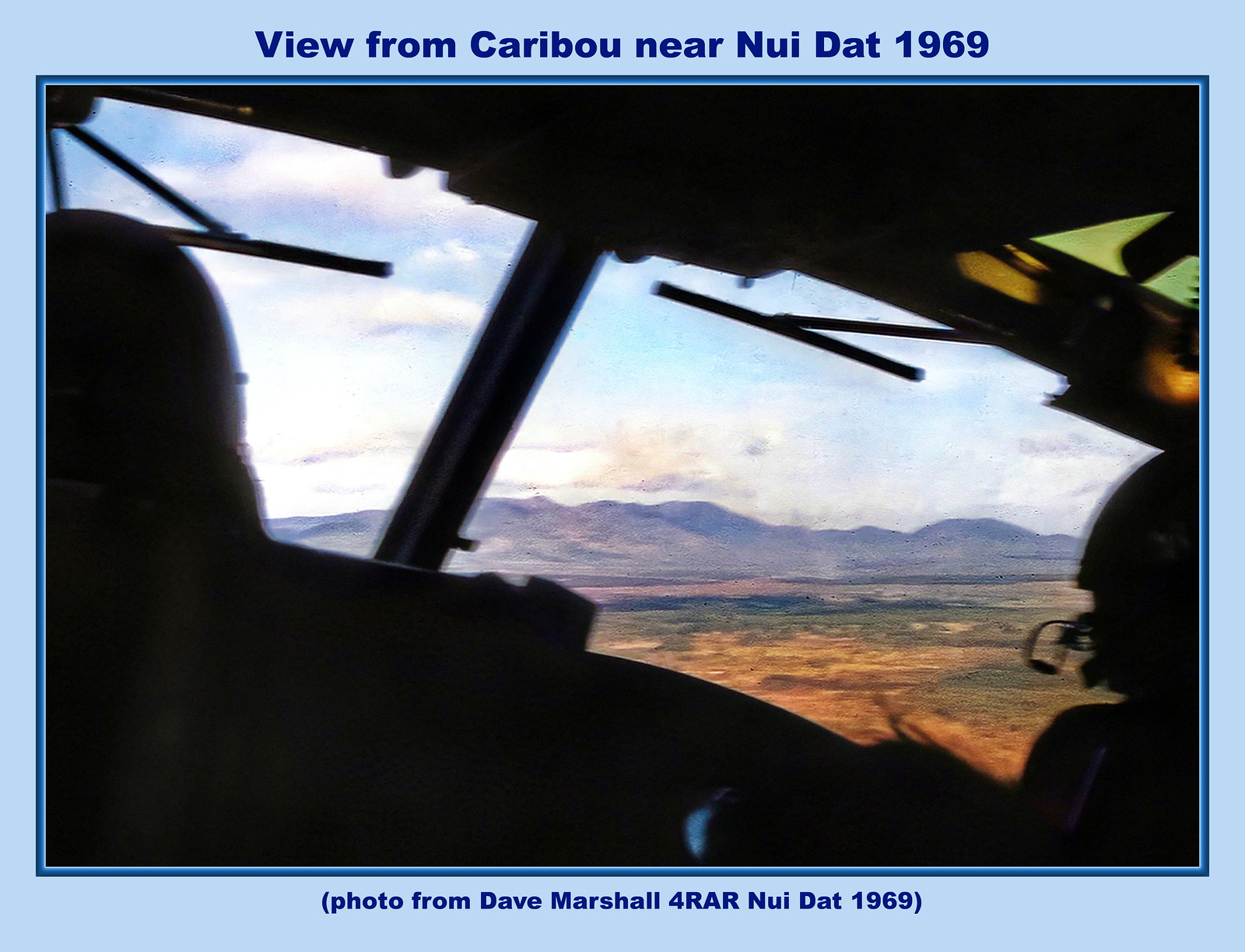The photograph, taken in 1969 near Nui Dat, Vietnam, is mounted with a darker blue rectangular outline and a lighter blue border. The title at the top, in dark blue font, reads "View from Caribou near Nui Dat, 1969." Below, it states, "(Photo from Dave Marshall for AR, Nui Dat, 1969)."

The image captures a slightly blurry but evocative scene from inside a military plane, likely a Caribou, with two pilots in view—one on the left and one on the right—wearing military helmets. The cockpit, dimly lit, features windshield wipers on the windows. Through the cockpit windows, an expansive landscape unfolds, revealing a rugged mountain range stretching across the horizon, with sparse grass and raw land in the foreground under a clear blue sky.